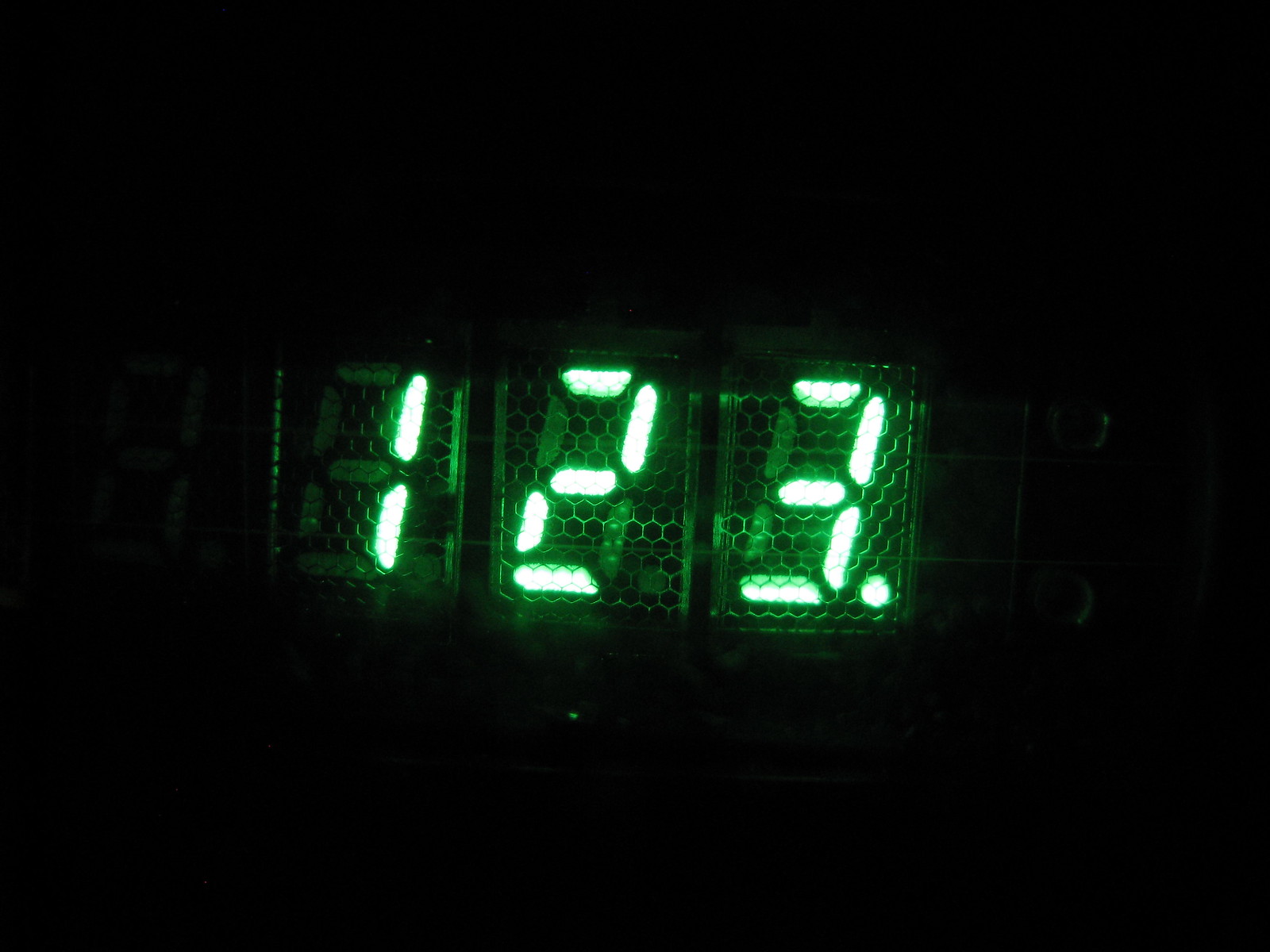The image features a digital screen against a completely black background, with three glowing digital numbers: 1, 2, and 3, followed by a decimal point. Each number is a neon green and appears within a square-shaped section, indicating some sort of display system. The numbers are centered in the middle of the image, and beneath the number 2, there's a small circle of green light. The display is constructed with a faint hexagonal grid pattern behind each number, formed by interlocking hexagons that are the same green color but dimmer. Additionally, three thin wires run horizontally across the screen in front of the numbers. While the exact purpose of the screen is unclear, it could be anything from a clock to a score counter or speedometer.